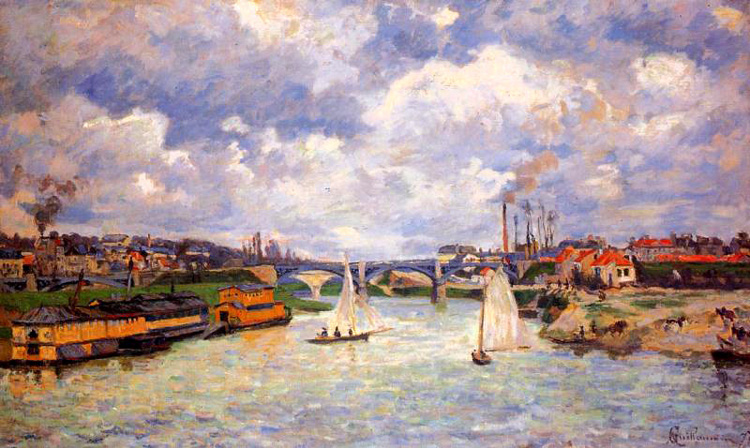This vibrant and detailed painting depicts a picturesque riverside scene, likely set in a European suburb or small city. In the middle of the image, a serene blue river flows gently, bisected by a blue bridge extending from one side to the other. The river is dotted with sailboats and large yellow boathouses with black roofs lining the left bank. On both sides of the river, charming houses with orange roofs and white or green walls cluster densely, adding to the quaint atmosphere.

The left side of the painting features a factory with a towering chimney emitting dark smoke, and a similar smoke stack rises from a large building on the right side. The surrounding area showcases a variety of architecture, with many large buildings in the background and a possible hillside terrain adding depth to the scene.

Notably, there are grazing animals on the right, contributing to the painting’s bucolic feel, and the tranquil river conditions are highlighted by the calm weather. The sky above is a brilliant blue, filled with an array of white clouds, casting a bright and lively light over the entire scene. Painted in a portrait orientation, this watercolor impressionist piece captures the serene beauty and bustling life of a riverine cityscape.